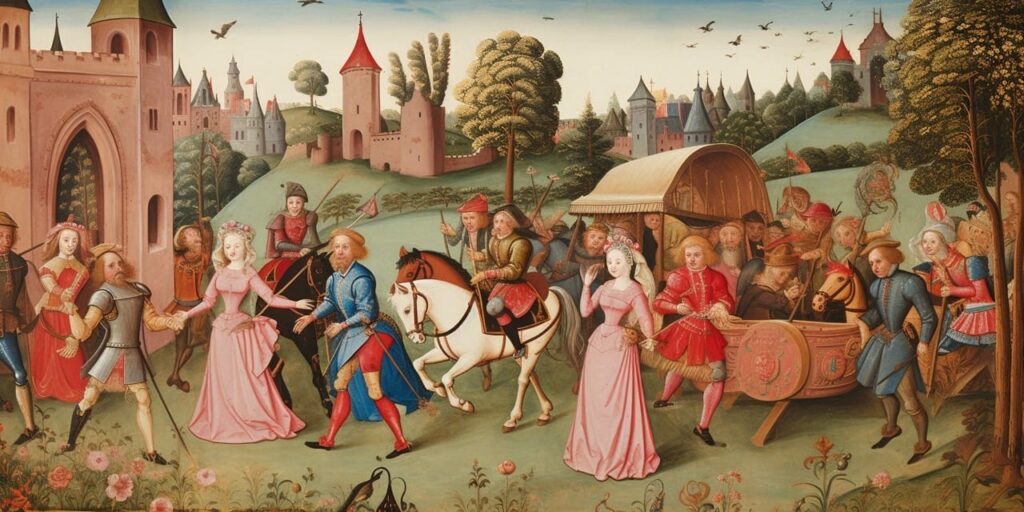The image depicts an elaborate renaissance or late medieval painting, teeming with vibrant activity against a backdrop of picturesque castles and lush green hills. In the foreground, a bustling crowd of people is captured in mid-procession, all headed primarily to the left. The women, adorned in flowing pink dresses cinched tightly at the waist by bodices, stand out with their headdresses draped with veils. Men in the scene wear tight breeches, stockings, and long overcoats that reach their knees. Several men are mounted on horses, and a few are seen riding in uniquely constructed carriages, some featuring pavilion-like coverings.

A noteworthy castle dominates the left side of the painting, with more castles scattered across the background, numbering up to five and varying in pink and blue hues. The sky above is a bright blue, dotted with birds in flight, adding to the sense of movement and liveliness. The entire scene is set outdoors amidst an array of trees with lush, green foliage, enhancing the vibrant, celebratory air of the painting.